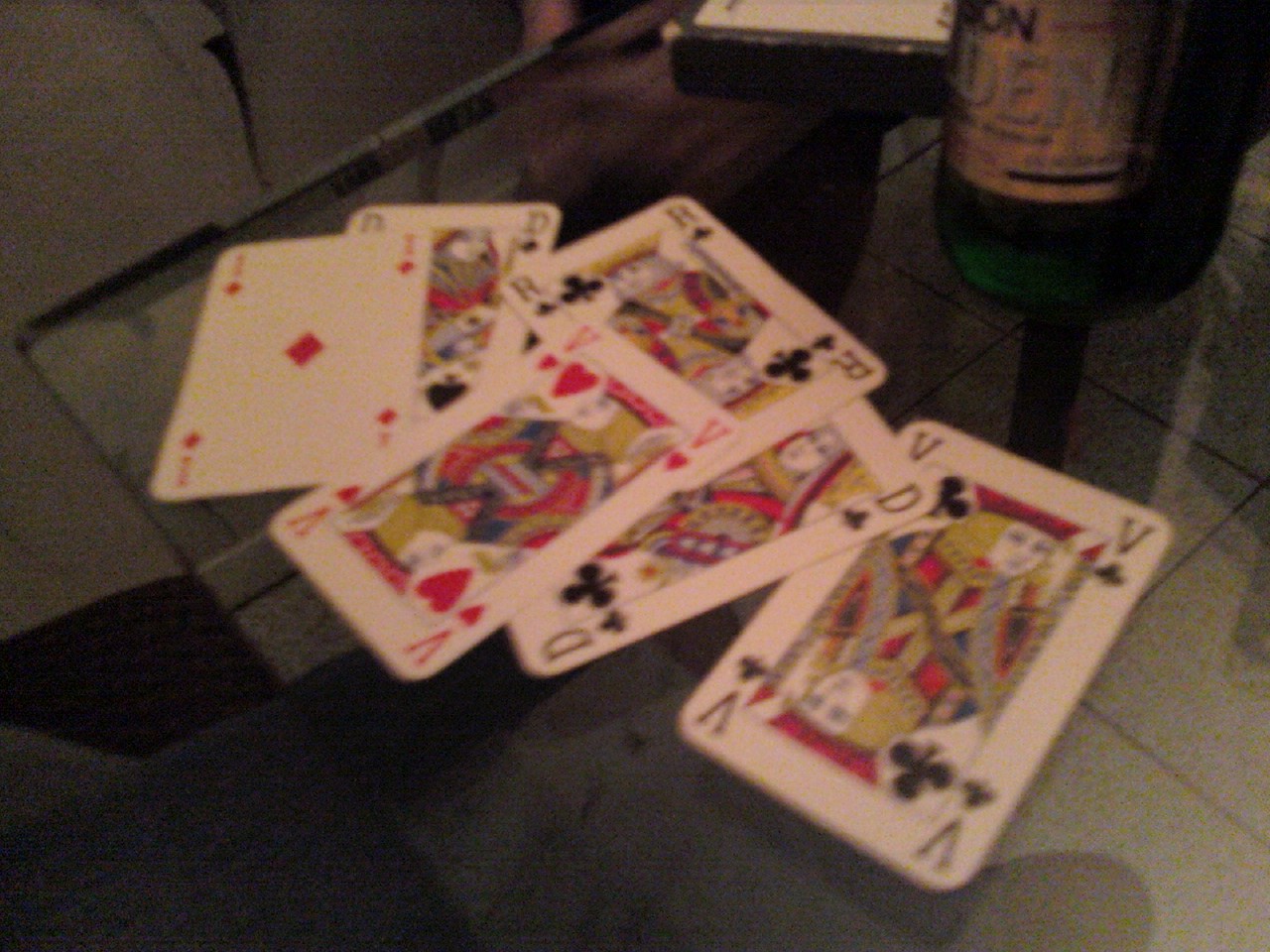The image features an assortment of six cards displayed on a table. Each card has unique and unusual markings, deviating from traditional playing card designs. 

- The first card, much like an ace, features a single diamond in the center and four smaller diamonds in the corners, but the symbolic value is unclear.
- Below it is a card that might represent a queen, depicted with a spade symbol.
- On the right is a card styled as a king of clubs; however, it is marked with the letter "R" instead of the standard "K."
- Adjacent to it is a jack of hearts, distinguished by the letter "V" replacing the customary "J."
- To the left, there is a card that appears to be a queen of clubs, marked with the letter "D."
- Lastly, there is another card resembling a jack of clubs, also marked with a "V."

This collection presents a peculiar arrangement of cards, each marked with atypical letters, challenging traditional expectations and raising curiosity about their origin or purpose.